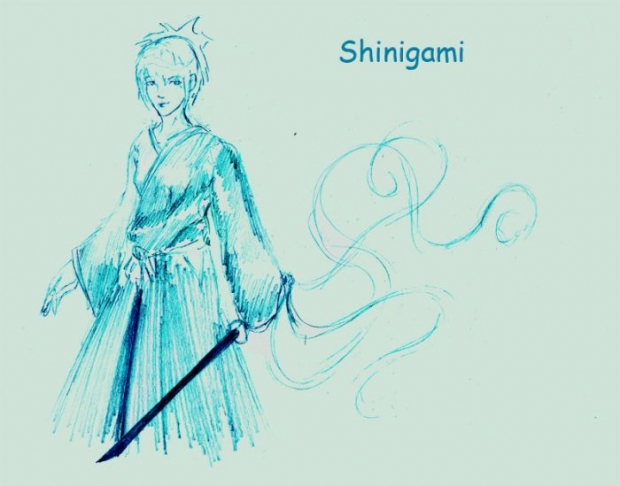In this artistic, hand-drawn image set against an olive green background, a person, possibly a female, stands towards the left side. The figure, depicted with spiky hair, is dressed in a robe-like outfit and a headband. They hold a long sword with trails or curlicue-like smoke designs extending from its end, giving the impression of recent movement. The sword is angled downwards in the person's left hand, while the right hand remains free. The drawing, done in shades of green, blue, and black with hints of off-white teal, carries a distinct anime feel. The only text in the image is "Shinigami," located in the upper right corner. The figure is in an upright position, facing slightly to the left but looking almost straight ahead.